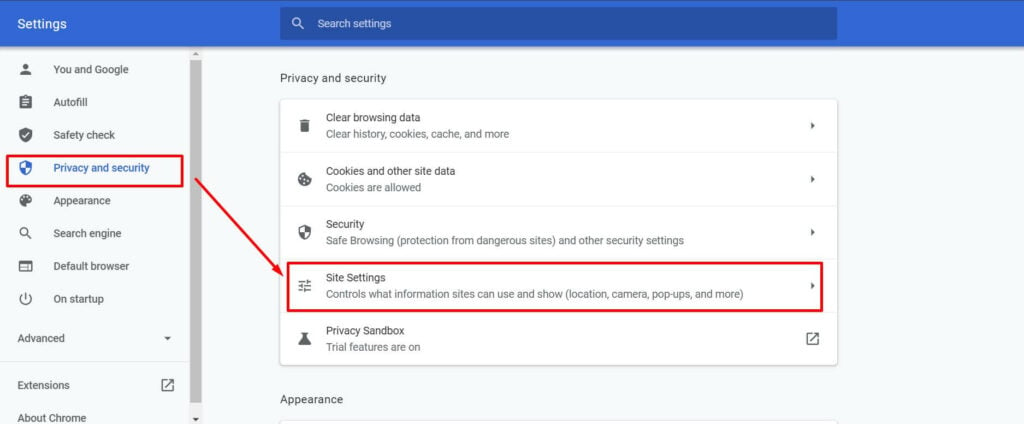The image depicts the settings page of Google Chrome. At the top left corner, "Settings" is prominently displayed in white text. Beneath this, a vertical menu lists various settings categories, each representing different configuration options. The listed categories include: "You and Google," "Autofill," "Safety Check," "Privacy and Security," "Appearance," "Search Engine," "Default Browser," "On Startup," followed by an "Advanced" dropdown button, "Extensions," and "About Chrome." The "Privacy and Security" section is highlighted in blue, indicating that it is the currently selected tab.

In the main section of the screen, "Privacy and Security" is the headline, followed by several options such as "Clear browsing data," "Cookies and other site data," "Security," "Site Settings," and "Privacy Sandbox." A red box outlines the "Site Settings" option, which includes a descriptive note: "Controls what information sites can use and show (location, camera, popups, and more)."